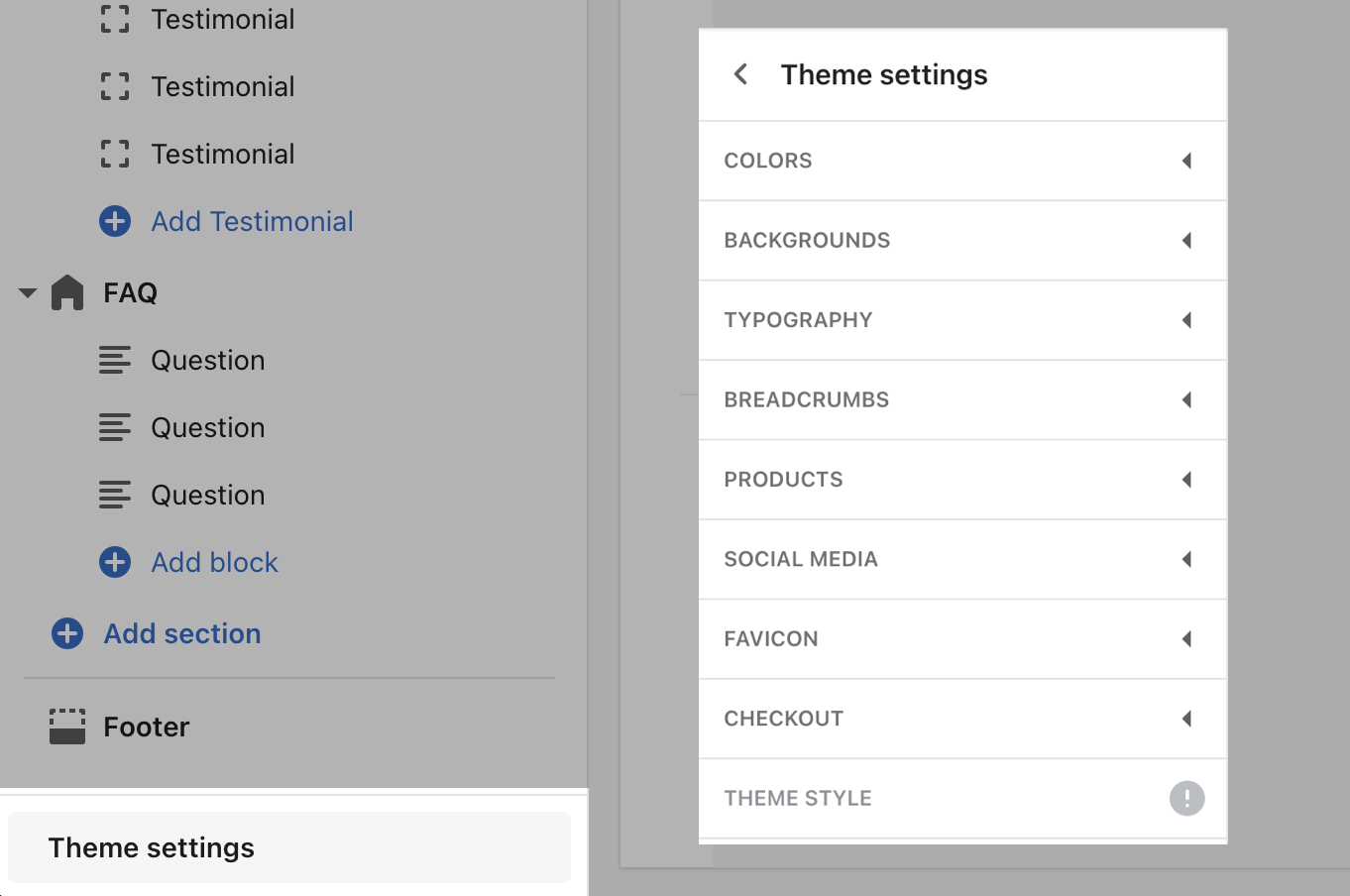The image depicts a horizontal user interface screenshot from a computer or smart device, seemingly of a settings menu. The background is slightly grayed out, accentuating the main focus on a prominent white pop-up box. 

On the left-hand side of the image, there are several textual elements in black. At the top, it reads "Testimonials" repeatedly, accompanied by a small square icon to the left. Below this, there is a blue plus sign that indicates "Add Testimonial." Further down, there are options labeled "FAQ," "Add Block," "Add Section," and "Footer." The bottom-most option is "Theme Settings."

On the right-hand side, the pop-up box obscures most of the background, but it's clear that the background is gray. Positioned at the top of the pop-up box is a bold black back arrow labeled "Theme Settings." Below this, the options are separated by lines with each option heading toward the right with an arrow icon indicating they can be expanded. The options listed are "Colors," "Backgrounds," "Typography," "Breadcrumbs," "Products," "Social Media," "Favicon," "Checkout," and "Theme Style." Notably, the "Theme Style" option is distinguished by a gray circle containing a white exclamation point.